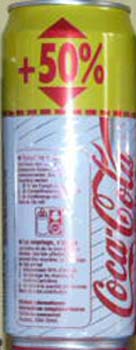On a pristine white background stands a striking aluminum can of Coca-Cola. The top of the can glistens with its silver finish, encircling the can's opening. Below the silver top, a yellow wrapping encompasses a section of the can, prominently featuring bold red arrows pointing up and down. Between the arrows, a message in vivid red letters reads "PLUS 50%". Beneath the yellow band, a slender red dotted line encircles the can, adding a touch of detail. The main body of the can showcases alternating white and silver stripes, creating a sleek pattern. Dominating the front of the can, the iconic Coca-Cola logo is emblazoned in rich red letters. On the side, the can provides comprehensive information on the ingredients and nutritional values. This elongated can of Coke commands attention with its vibrant design and detailed labeling.